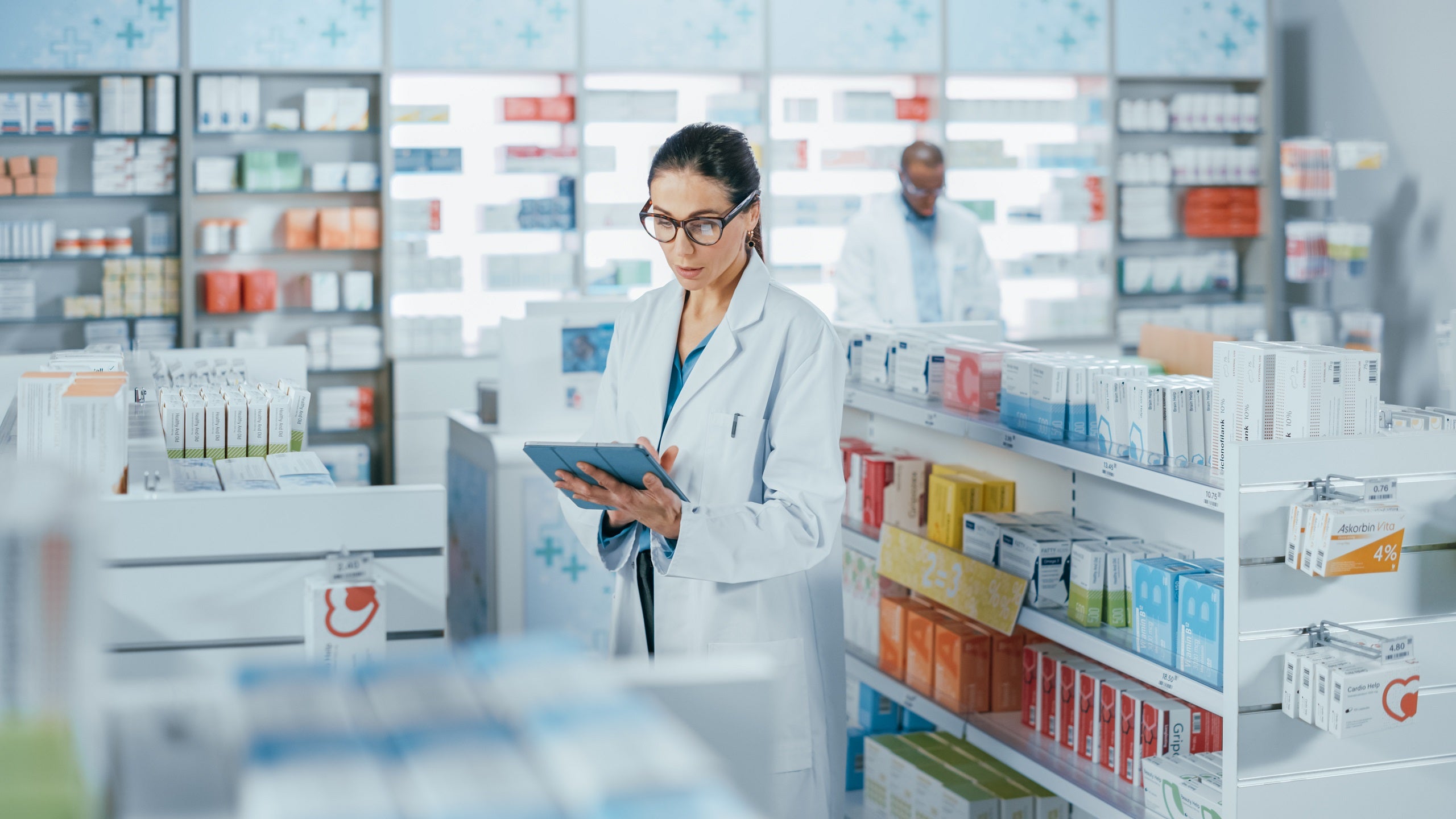In this image of a pharmacy, white dominates the color palette, with white shelves, counters, computers, cupboards, and walls. The top of the image features white signs adorned with turquoise plus symbols, casting a sterile, clinical atmosphere. Beneath these signs, illuminated shelves are lined with various boxes and jars of medications, organized meticulously.

The foreground showcases a female pharmacist engrossed in her task. She has black-framed prescription glasses and slicked-back black hair, dressed in a white lab coat over a blue or green undershirt. With a focused expression, she holds a tablet in her left hand, seemingly doing inventory or taking notes.

In the background, another pharmacist, a Black gentleman with glasses, mirrors her attire with a white lab coat and a blue shirt. He is concentrated on a task that remains obscured by the shelves, adding depth and busyness to the scene. This image vividly captures the meticulous and organized environment of a modern pharmacy, highlighting the pharmacists' dedication to their responsibilities.